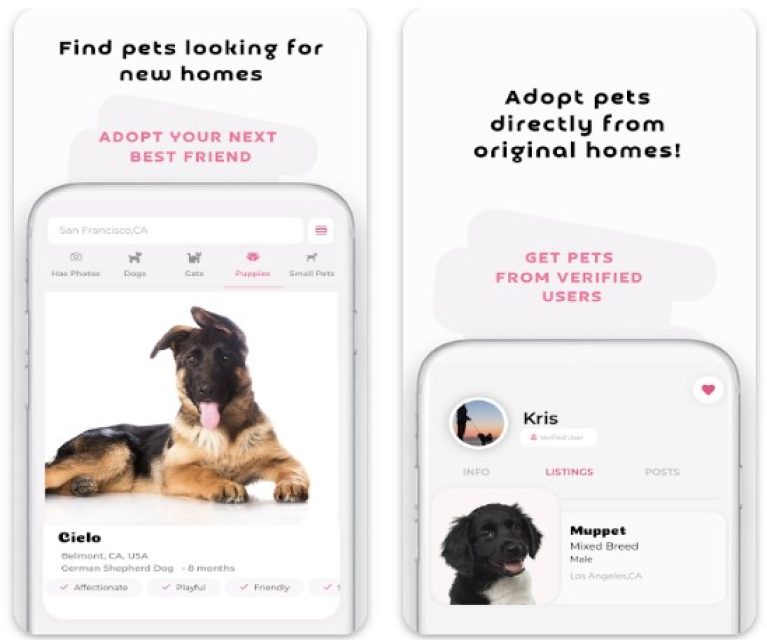The image is divided into two distinct sections. 

**Left Side Description:**
- In the center of the left side, there is a black text that reads: "Find pets looking for new homes."
- Below this text, there is a pink text that says: "Adopt your best friend."
- An illustration of a cell phone's exterior is prominently displayed. On its screen, the search bar shows: "San Francisco, CA."
- Beneath the search bar, gray text reads: "Has photos."
- Following this, there are silhouette images of different animals: a small dog, a cat labeled "Cats," and "Small pets" on the far right side.
- In pink text, the word "Puppies" is highlighted.

- Below this, there is an image of a German Shepherd dog. The dog has a black face, its tongue sticking out, and one ear folded over the other, with the unfolded ear pointing left. The dog is lying down with its front paws stretched out.
- The dog’s name "Celio" is written in black, with further details provided: "California, German Shepherd dog, eight months."

**Right Side Description:**
- Black text at the top right reads: "Adopt pets directly from original homes."
- Below this, pink text says: "Get pets from verified users."
- An outline of a cell phone is shown, with a profile picture of a person holding a dog on a leash.
- Beside this, the name "Chris (K-R-I-S)" is displayed.
- Below Chris's profile, there is an image of a dog with black fur and a patch of white fur. The dog's mouth is slightly open.
- The dog's details are given: "Muppet, mixed breed male."

This detailed descriptive caption for the image provides a clear understanding of its content, presenting the visuals and textual elements in a coherent manner.